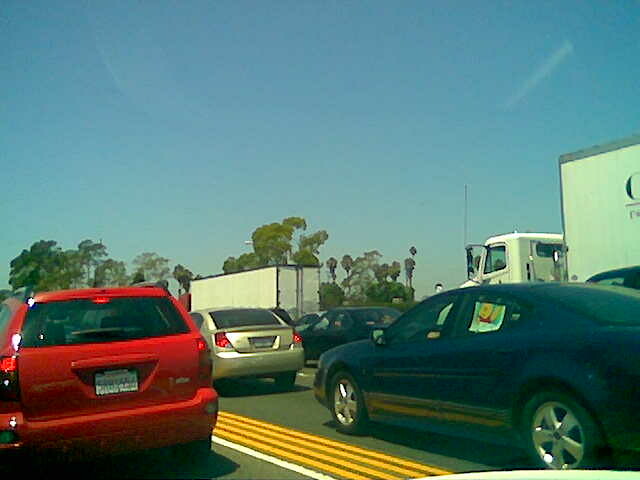This slightly blurred photograph captures a crammed roadway scene, likely from bumper-to-bumper traffic, taken from within a vehicle either in the passenger or driver’s seat. The photo shows four lanes of cars lined up one behind the other, illustrating a significant traffic jam. The leftmost lane has a triple yellow line to the right of it, indicating it might be a designated carpool lane.

In the foreground, directly in front of the photographer’s vehicle, there's a red station wagon. To its right in the neighboring lane, there's a gold sedan, possibly an early 2000s Saturn, followed by a blue sedan with a children's icon, likely Winnie the Pooh, affixed to the back window, suggesting the presence of children. Further right, in the far lane, are large white tractor trailers, with one positioned behind a dark-colored vehicle, likely signaling the slow lane designated for large trucks.

Tall trees peak above the tops of these vehicles against a backdrop of clear blue sky with faint streaks of clouds, adding a touch of tranquility to the otherwise congested scene.